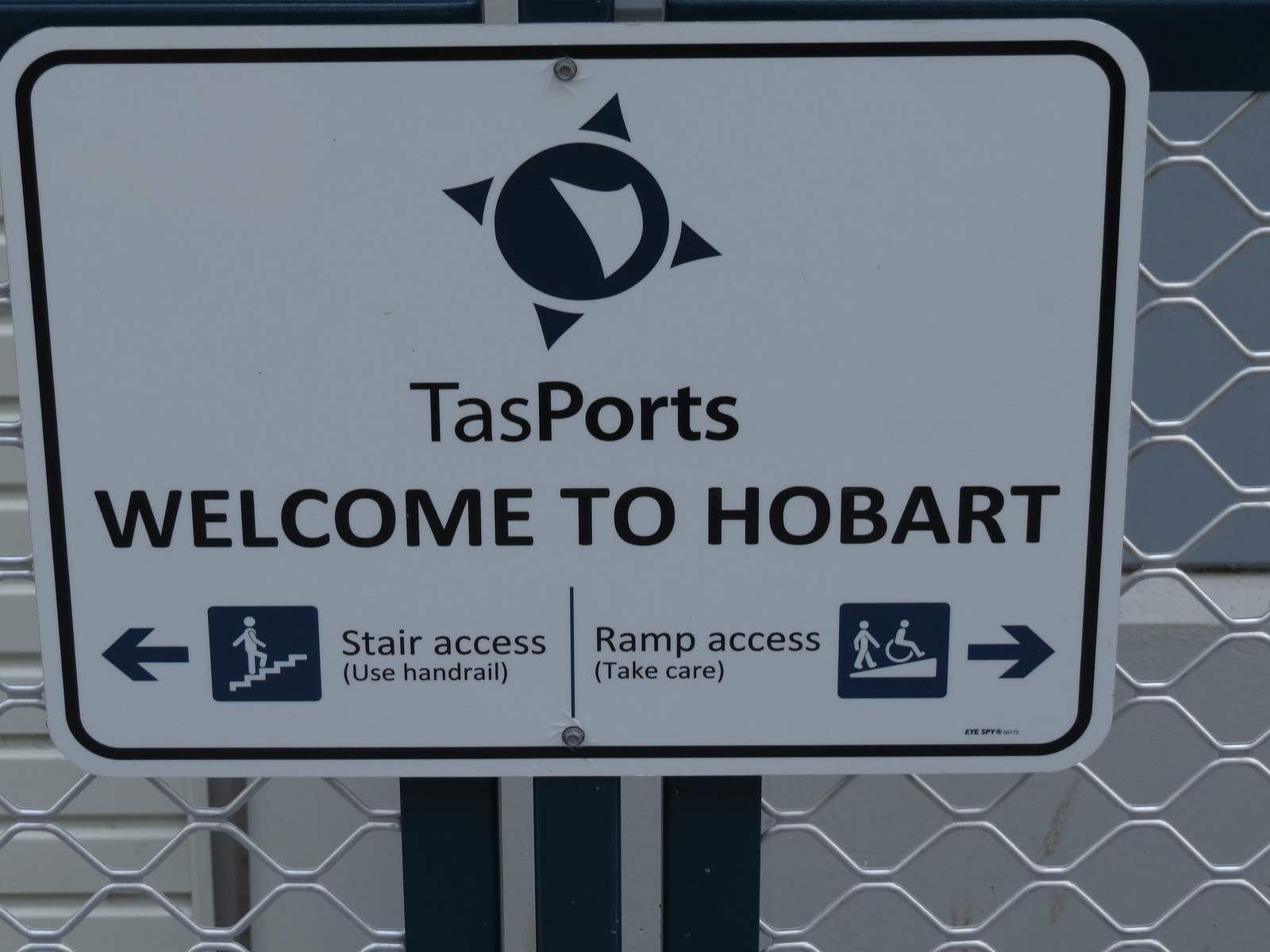The image depicts a rectangular white sign mounted on a white linked fence. The top half of the sign features a black circle overlaid by four black triangles pointing slightly diagonally, indicating compass points with the top one positioned between 12 and 1 on a clock face. Inside the circle, there's a curved triangle pointing to the top-left, suggesting dynamic motion. 

Below this logo, the text "TASPORTS" is prominently displayed, followed by "WELCOME TO HOBART" in all capital letters. A dividing line separates the main text from the directional instructions below. 

On the left side, an arrow points left toward an icon of a person walking up a staircase with the directive "STAIR ACCESS, USE HANDRAIL." On the right side, another arrow points right toward an icon showing a person following another person in a wheelchair, indicating "RAMP ACCESS, TAKE CARE" (with "TAKE CARE" in brackets). 

The detailed elements, such as the black and white color scheme and the fencing in the background, contribute to the overall contextual setting of the sign as an informative guide at a port, specifically welcoming visitors to Hobart, Tasmania.